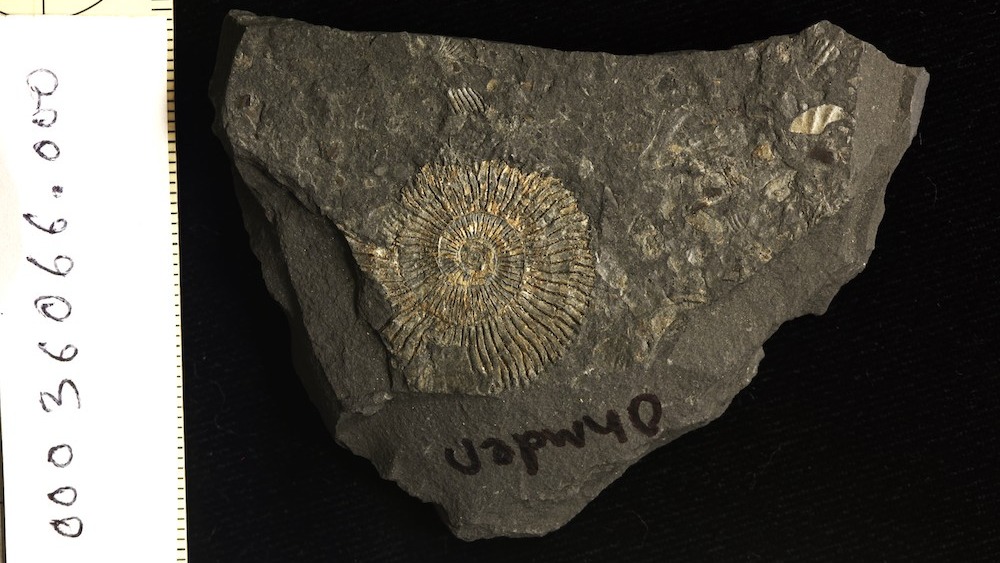The photograph depicts a large, dark gray, roughly triangular rock with a fossilized shell embedded in it, all set against a black background. The sides of the rock taper inwards but do not meet at a sharp point, suggesting it has been chipped or broken at the bottom. Dominating the central area of the rock is a prominent, circular fossil with a beige, spiral pattern that loops inward, resembling a mollusk or shell. The fossil appears ancient and weathered, with hints of beige and lighter colors interspersed throughout the rock’s gray surface.

On the rock, there is some illegible black ink writing that appears upside down, potentially spelling OHMDAN or OHMTEN. To the left of the rock, there is a white piece of paper displaying the vertically arranged numbers 0036066.000, which could indicate an identification or catalog number.